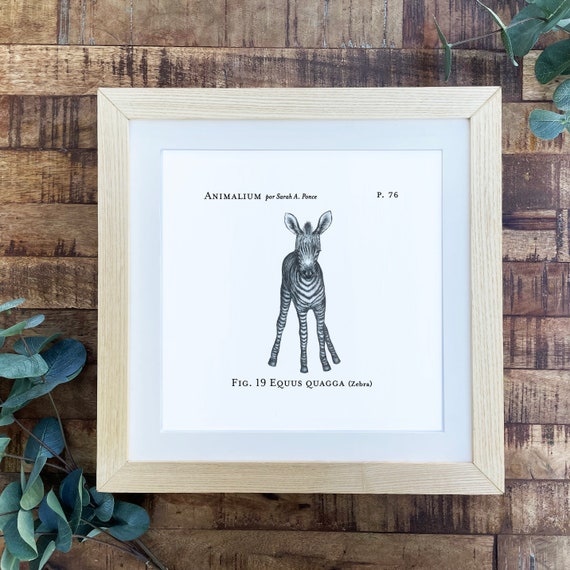The image showcases a quaint, rustic scene with a nostalgic charm. At its center is a framed illustration of a young zebra, meticulously rendered in black and white, set against a white background. This tasteful drawing, likely a pencil sketch, is encased in a light wooden frame complemented by a blue mat. The frame measures approximately 10 inches by 10 inches and is positioned against what appears to be the weathered wooden exterior of a house or shed, composed of old strips of wood. 

The illustrated zebra, with alert ears and distinct markings, gazes directly towards the viewer. The text above the zebra reads "Animalium Porcera a Ponce," and directly below it, the label "Fig. 19 Equus Quagga (zebra)" is inscribed, along with a page reference "P.76," indicating this image was likely extracted from a textbook or scientific publication. Adding a touch of nature, dark green leaves partially frame the image, appearing prominently in the upper right and bottom left corners of the shot.